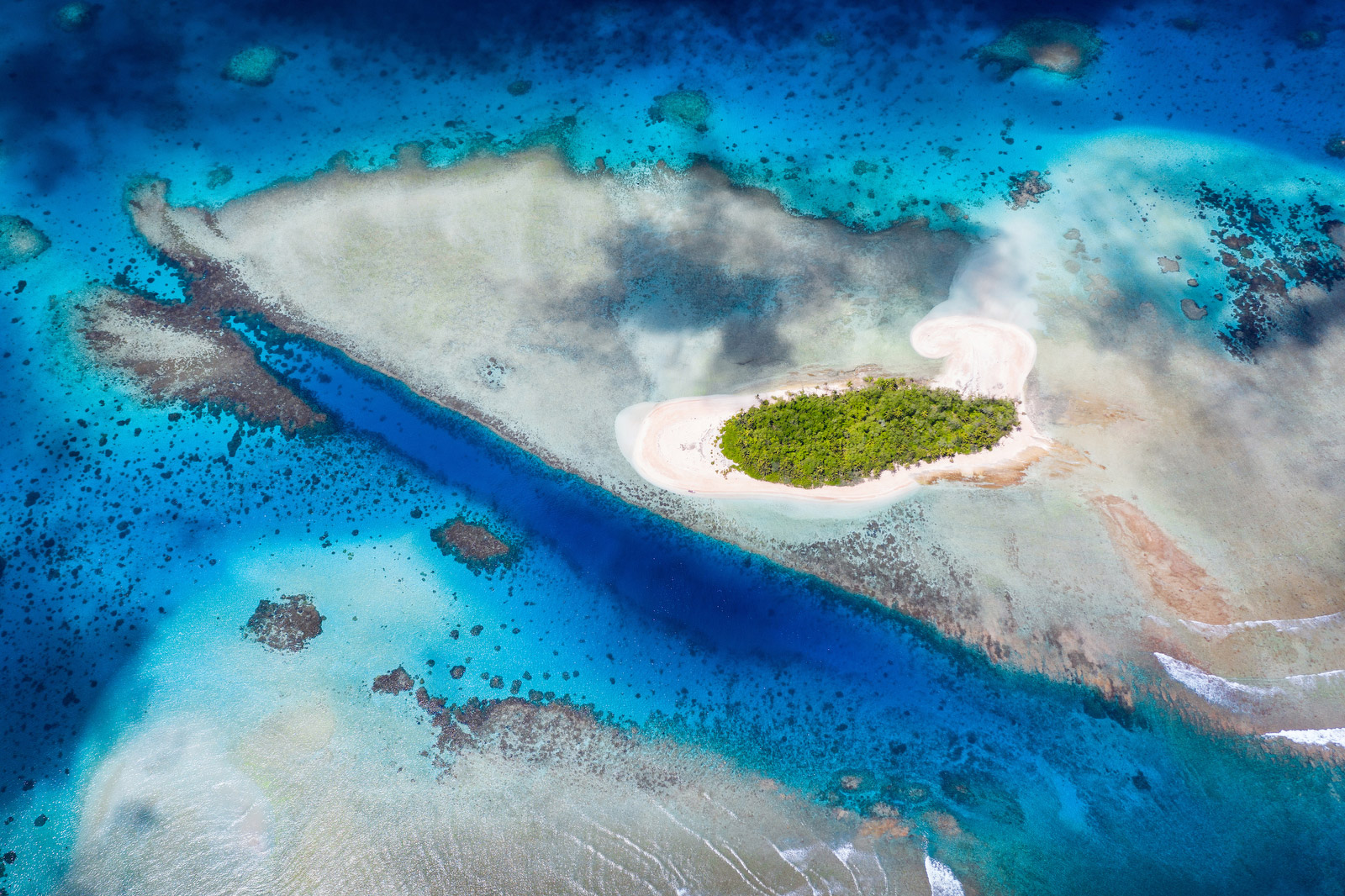The aerial photograph showcases a vibrant waterway with multiple shades of rich blue hues, including turquoise and royal blue. The clarity of the water reveals speckles throughout, and at the bottom, shallow regions featuring small raised areas and coral-like formations. Dominating the scene is a lush green island with fluffy treetops and dark gray speckles scattered across its surface. The island is surrounded by a contrasting shoreline of pinkish light tan sand, creating a distinct border against the water. Additional unfocused areas suggest varied depths and possibly specialized imaging to highlight these nuances, making the scene both captivating and detailed.